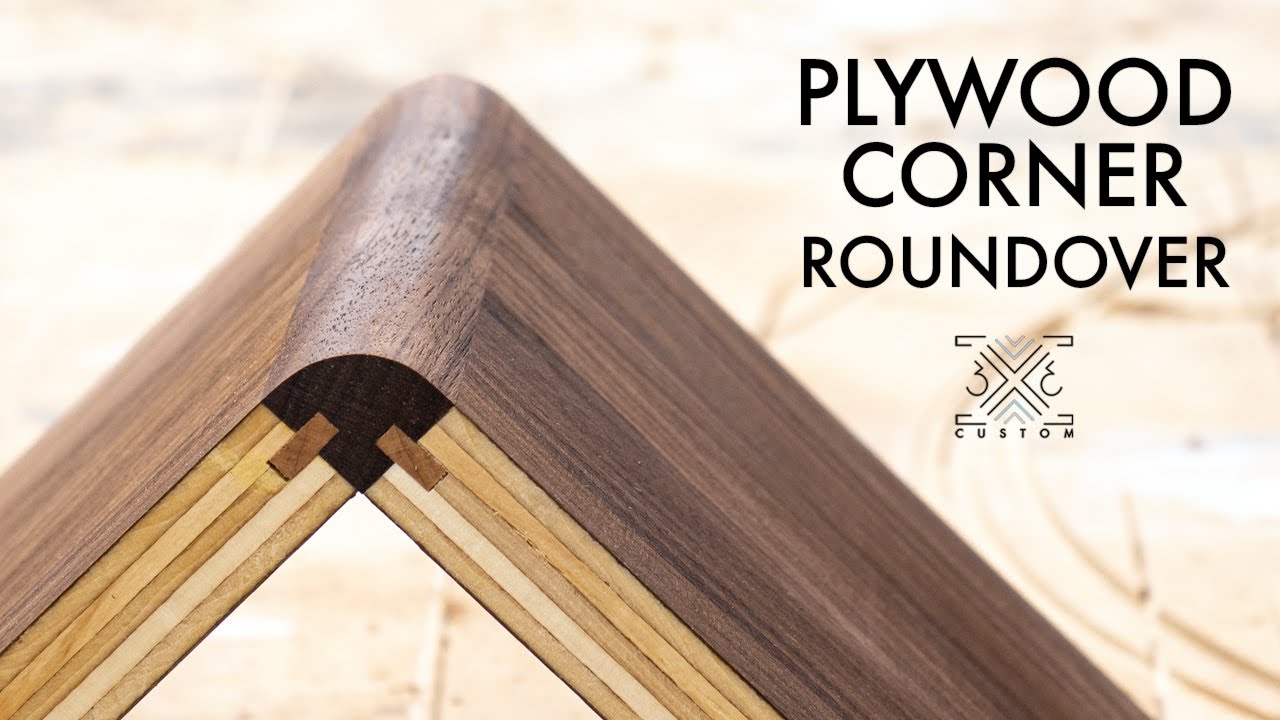The image is an advertisement for a woodworking technique featured in a rectangular frame, approximately five to six inches wide and three inches high. The background consists of a very light beige color, subtly blending into white with faint coffee stains or edges visible, and includes a small black stain in the upper left corner. Dominating the lower left-hand corner and extending upwards at an angle is a precisely detailed wooden corner. This corner appears to be crafted from one solid piece of dark-stained wood, likely walnut, smoothly rounded without sharp edges. The wood is constructed from five-ply thin layers, each glued together with varying shades of beige, yellow, brown, and gold, presenting a visually appealing multi-tonal effect. At the top right of the image, there is a caption in black print reading "PLYWOOD CORNER ROUNDOVER," with the word "CUSTOM" in all capital letters directly beneath it. This descriptive visualization aims to highlight the craft and custom design of the plywood corner roundover, ideal for woodworking enthusiasts or professionals.